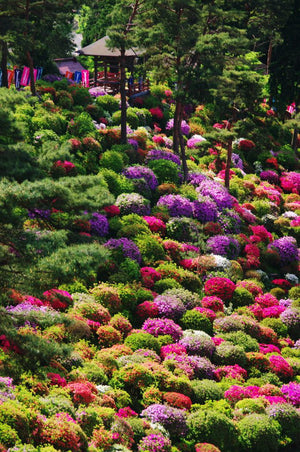This vibrant landscape photograph captures a meticulously manicured hillside adorned with an array of colorful flowering bushes. The well-tended shrubs, predominantly circular and bushy in shape, cover the slope in a stunning tapestry of colors—ranging from greens and yellows to vivid shades of pink, magenta, purple, and even multicolored varieties. Interspersed among the flowering plants are patches of green ornamental grasses and additional shrubs, contributing to the lush scenery. Further up the hill and dotted sporadically are taller, straight vertical trees with a rich, dark green foliage.

In the background of this serene scene stands a small, circular-roofed hut, identifiable as an Asian-style gazebo or tea house. This charming structure is surrounded by dark green trees and flanked by pink flags and colorful banners that hang along the walkways, matching the vibrant hues of the floral display. The overall image exudes an air of tranquility and careful cultivation, with every element thoughtfully placed to create a picturesque and serene natural setting.